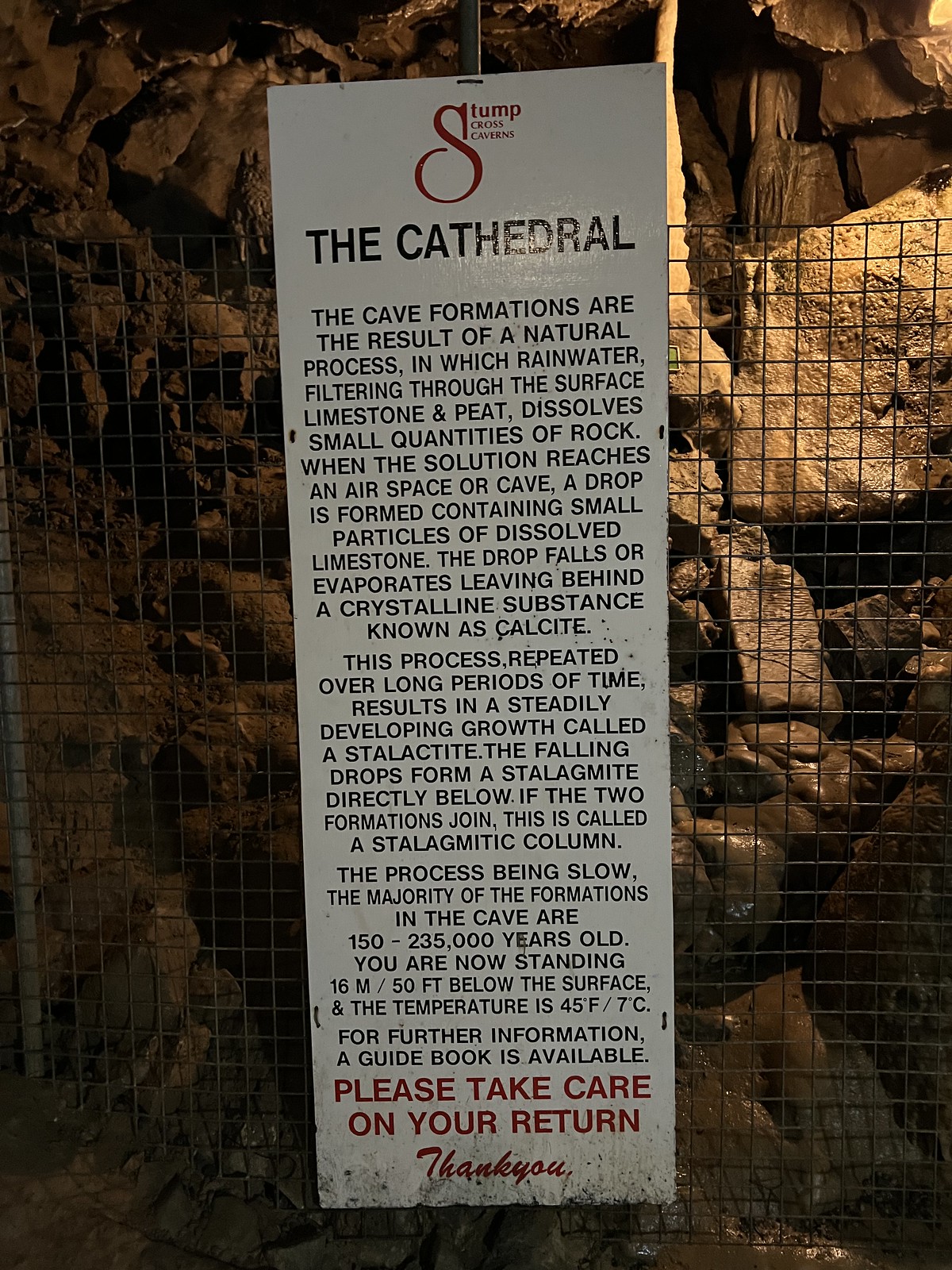The photograph depicts the entrance to a cave known as Stump Cross Caverns. It features a rock wall comprised of stacked and crumbled rocks, which is protected by a wire safety mesh. A prominent white sign with bold red and black text reads "Stump Cross Cavern" and "The Cathedral," marking the entrance to the Cathedral Room. Informational text on the sign explains that the cave formations result from a natural process where rainwater filters through surface limestone and peat, dissolving small quantities of rock. When the solution reaches an airspace or cave, it forms drops containing dissolved limestone particles that eventually deposit calcite as the drop falls or evaporates. Over long periods, this slow process creates stalactites from the ceiling and stalagmites on the ground. If these formations eventually join, they form a stalagmitic column. Most of the formations in this cave are approximately 150,000 to 235,000 years old. Visitors stand 50 feet (16 meters) below the surface, where the temperature is a constant 45 degrees Fahrenheit (7 degrees Celsius). A guidebook is available for further information, and visitors are advised to take care on their return.